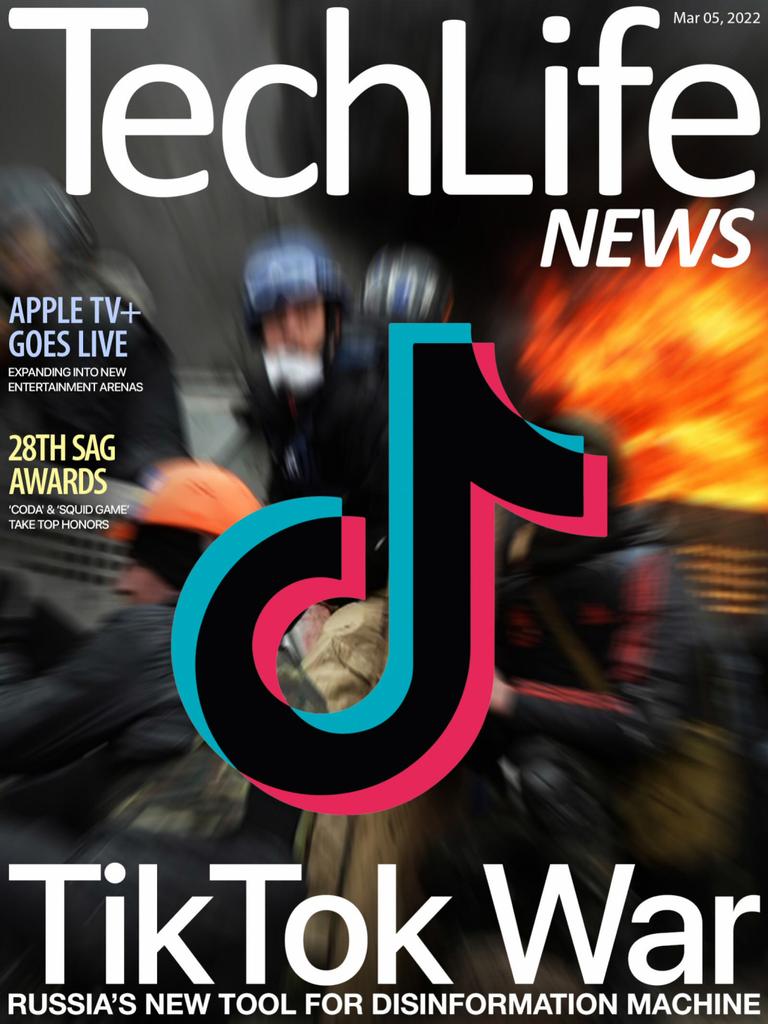**Tech Life Magazine - March 5, 2022 Edition**

On the cover of the latest issue of Tech Life Magazine, the title "Tech Life" is prominently displayed in large white print across the top. Adjacent to the title, in smaller print, the publication date of March 5, 2022, is noted alongside the subtitle "Tech Life News."

The background of the cover features a dramatic and somewhat enigmatic image, resembling a figure in a motorcycle helmet surrounded by flames, creating an ominous and intense atmosphere that suggests a sense of movement and action.

On the left-hand side of the cover, two featured articles are highlighted:
1. **Apple TV Plus Goes Live** - Expanding into new entertainment arenas.
2. **28 SAG Awards** - CODA and Squid Game take top honors.

Dominating the center of the cover, the TikTok logo is prominently displayed, taking up approximately 25% of the page. The logo's distinctive black, blue, and red colors stand out.

Beneath the logo, in very large white print, the headline "TikTok WAR" captures attention. Directly below, a striking banner reads, "RUSSIA'S NEW TOOL FOR DISINFORMATION MACHINE," emphasizing the cover story's focus on the role of TikTok in spreading misinformation amid geopolitical tensions. The headline "TikTok WAR" is styled with a capital T, capital T, and capital W for emphasis.